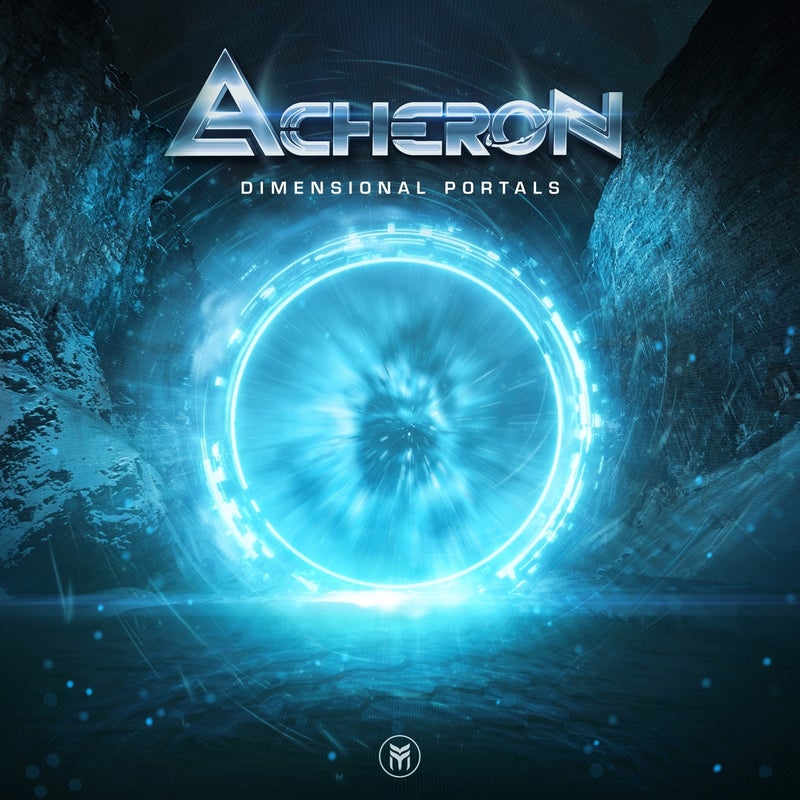The image evokes a vivid science fiction theme, resembling a movie poster, video game artwork, or an album cover. At its core, a radiant, teal-colored sphere or portal dominates the scene, casting a mesmerizing blue glow that intensifies towards the center before fading into darker shades along the edges. Encircling this luminous orb, rugged, rocky walls with blue snow-covered mountains are visible, contrasting the bright sphere's glow with their darker hues. The lower part of the image depicts a deep blue body of water, subtly reflecting the portal's ethereal light. 

Prominently placed at the top of the image, the word "ASHERON" (spelled A-C-H-E-R-O-N) stands out in a sparkly silver font, with the letter "O" uniquely encased in a surrounding ring reminiscent of a planetary orbit. Directly below this title, "Dimensional Portals" is inscribed in plain, white, all-capital letters. The overall composition features dark blue tones in the upper corners and speckles of varying blue shades near the bottom, adding depth to the scenery. Centered at the bottom of the image is an emblem or logo, featuring a stylized "M" encircled by a ring.

The visual presentation, rich in detail and brimming with a luminous blue-and-white color palette, suggests the gateway to another realm, perfectly capturing the essence of its mystical and futuristic theme.